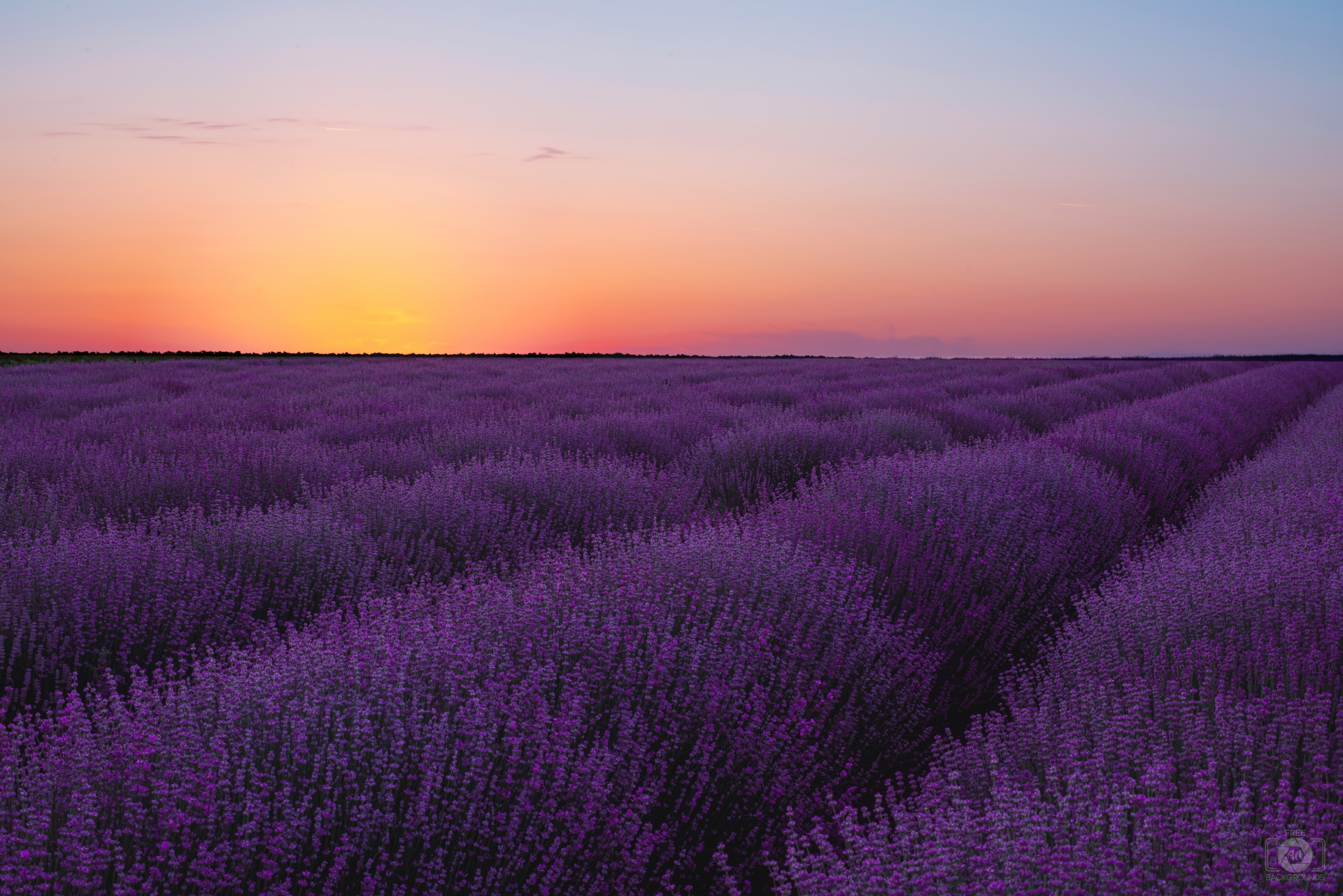The image depicts a breathtaking, endless field of lavender-like purple flowers, arranged in rows that stretch horizontally and vertically towards the horizon. The flowers, appearing as dense, shrub-like clusters, create a sea of purple that seems to go on forever. The sky above is mostly clear, with a few clouds lingering to the left, and a beautifully vivid sunset at the bottom right, casting an orange and yellow glow across the sky. The sun itself is partially hidden as it sets on the horizon, which is lined with a distant row of trees and possibly some mountains in the background. The overall scene is one of serene natural beauty, with the contrasting colors of the purple flowers and the warm hues of the setting sun creating a captivating visual.